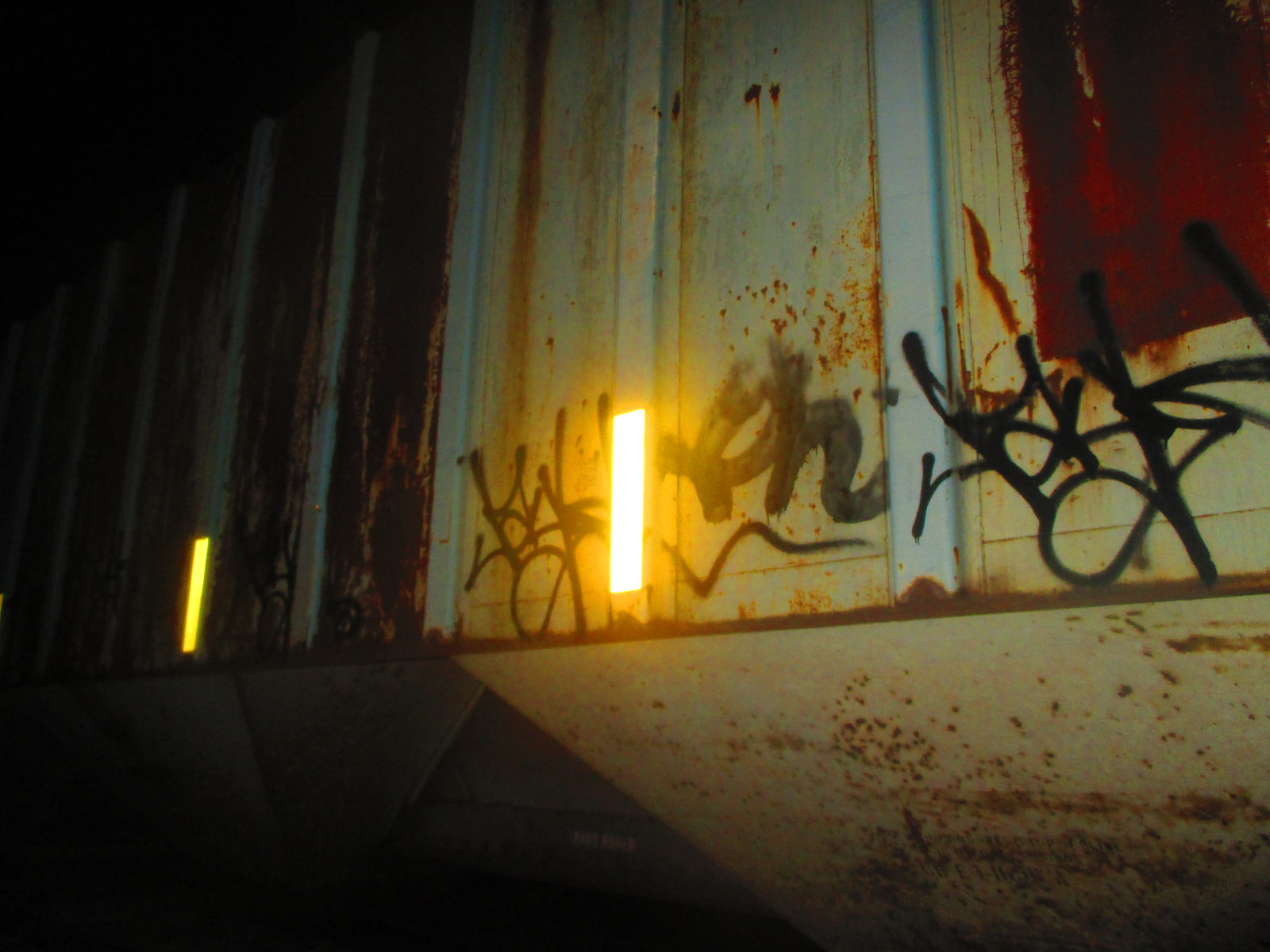In this nighttime outdoor scene, the left portion of the image is enveloped in pitch darkness. Toward the center and right, there's a segmented white metal wall, heavily rusted with numerous rust spots both at the top and underneath. The wall is intersected by white beams that also show signs of rust. Prominently in the middle beam, there's a bright rectangular light, possibly a reflection. An additional, dimmer light with a yellowish tinge can be observed on the left edge. The upper right-hand corner features a patch of red paint. Along the lower middle section, thick black graffiti marks, more like abstract squiggles than readable words, are visible. The rust appears heavier on the left side of the wall compared to the right side. A shadow is cast toward the bottom left, enhancing the contrast between the illuminated wall and the darkness surrounding it.